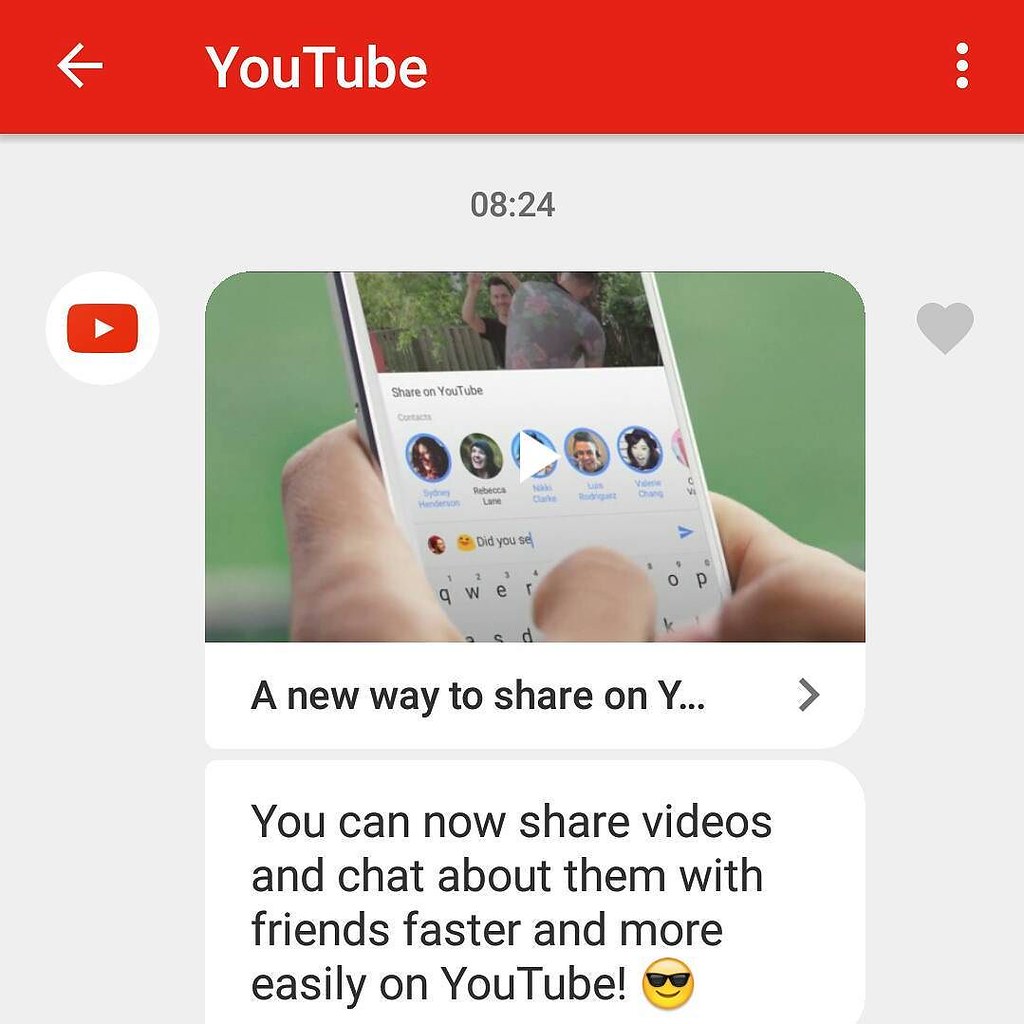This image is a screenshot of a YouTube interface highlighting a new messaging service. At the top of the screenshot, there is a video thumbnail featuring an individual holding a phone, displaying a YouTube video being shared. The video's title reads "Share on YouTube." Beneath this, there are profile pictures of various users with chat bubbles displaying their names. An on-screen keyboard is partially visible at the bottom, with a user in the process of typing the phrase, "Did you see..." accompanied by an Apple-style smiley face emoji. Further down, there is a notification banner with a message stating, "A new way to share on YouTube" followed by an arrow pointing down. Below this, the message continues to explain, "You can now share videos and chat about them with friends faster and more easily on YouTube." The banner concludes with a smiley face emoji wearing sunglasses.